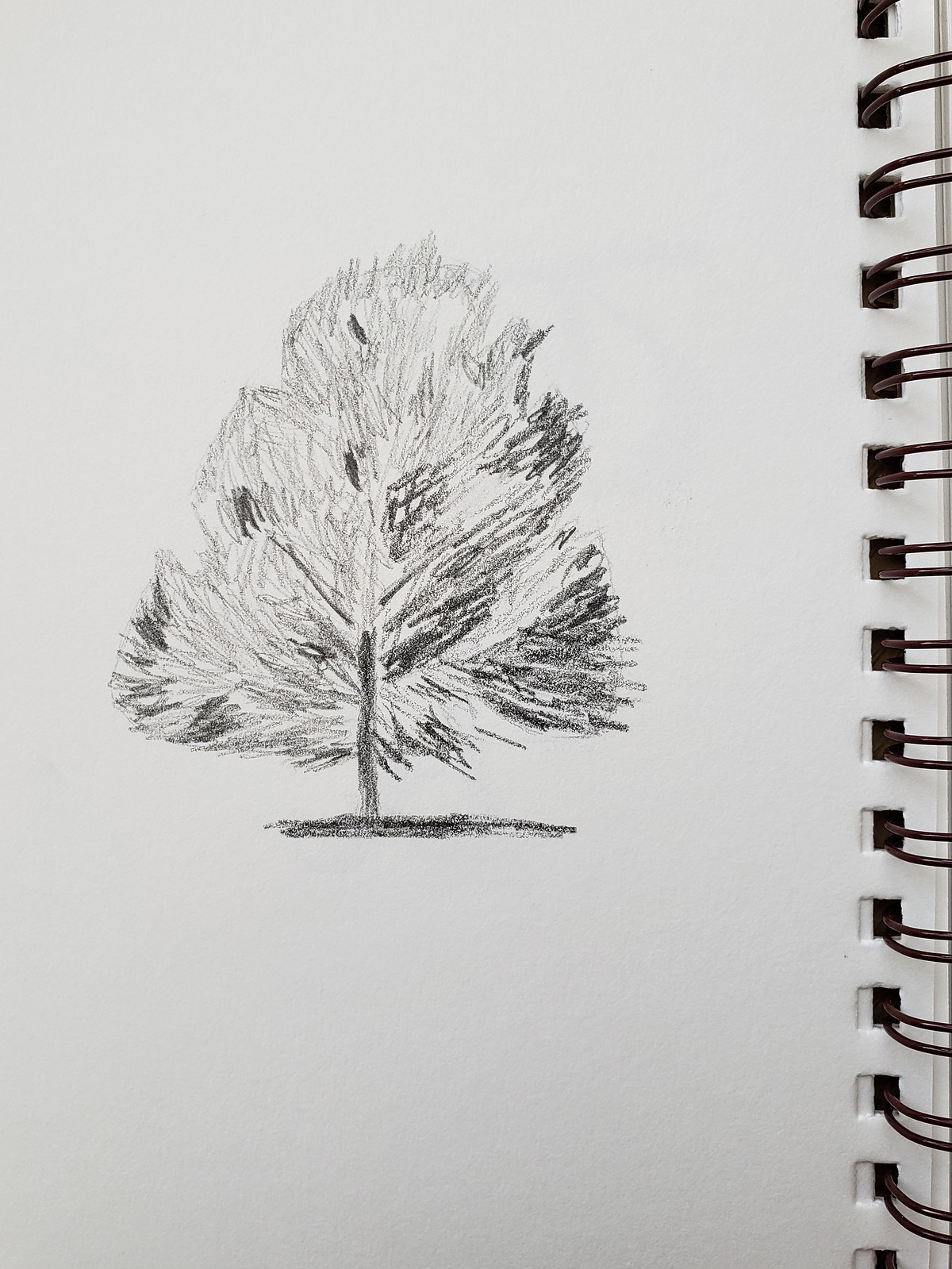The photograph showcases an open sketchbook, with emphasis on the left page. Visible to the right edge of the image is the black metal spiral binding of the sketchbook. Dominating the left page is a meticulously detailed drawing of a large tree, rendered in black pencil. The tree has a somewhat triangular shape, though its corners and edges are smoothly rounded, giving it a natural, flowing appearance. A shadow, cast by the tree, extends underneath it to the right, adding depth and dimension to the drawing. The image orientation is taller than it is wide, creating a sense of verticality and grandeur. There are no written annotations, no people, animals, buildings, or motorized vehicles in the illustration, emphasizing the solitary elegance of the tree.